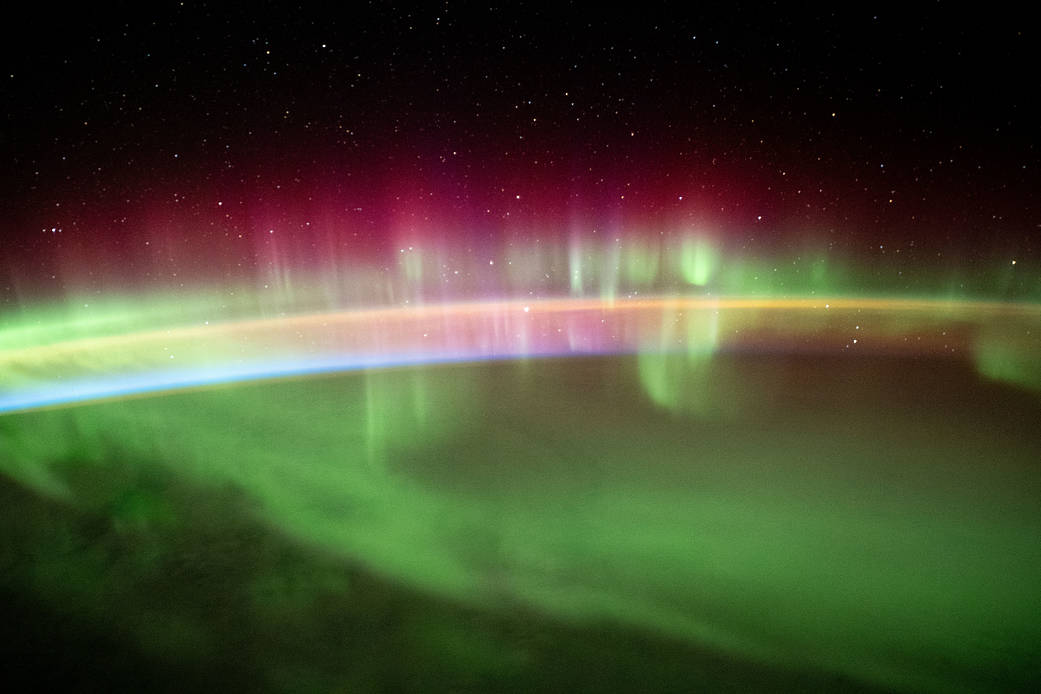This image captures the mesmerizing Aurora Borealis, possibly taken from an aerial or space view. The background is a pitch-black night sky punctuated with numerous twinkling stars, providing a sharp contrast to the blurred aurora in the foreground. The aurora features a dazzling, out-of-focus display of vibrant colors. At the top, shades of magenta and pink blend seamlessly into various hues of green, accented with a hint of yellow. These colors stretch vertically, resembling rays beaming upwards out of an arc. The bottom half predominantly showcases the dynamic, swirling greens characteristic of the aurora, mimicking what one might see while gazing up at this natural phenomenon from Earth. The ethereal swirl of cosmic rays and the gradient of colors accentuate the celestial beauty of the scene.